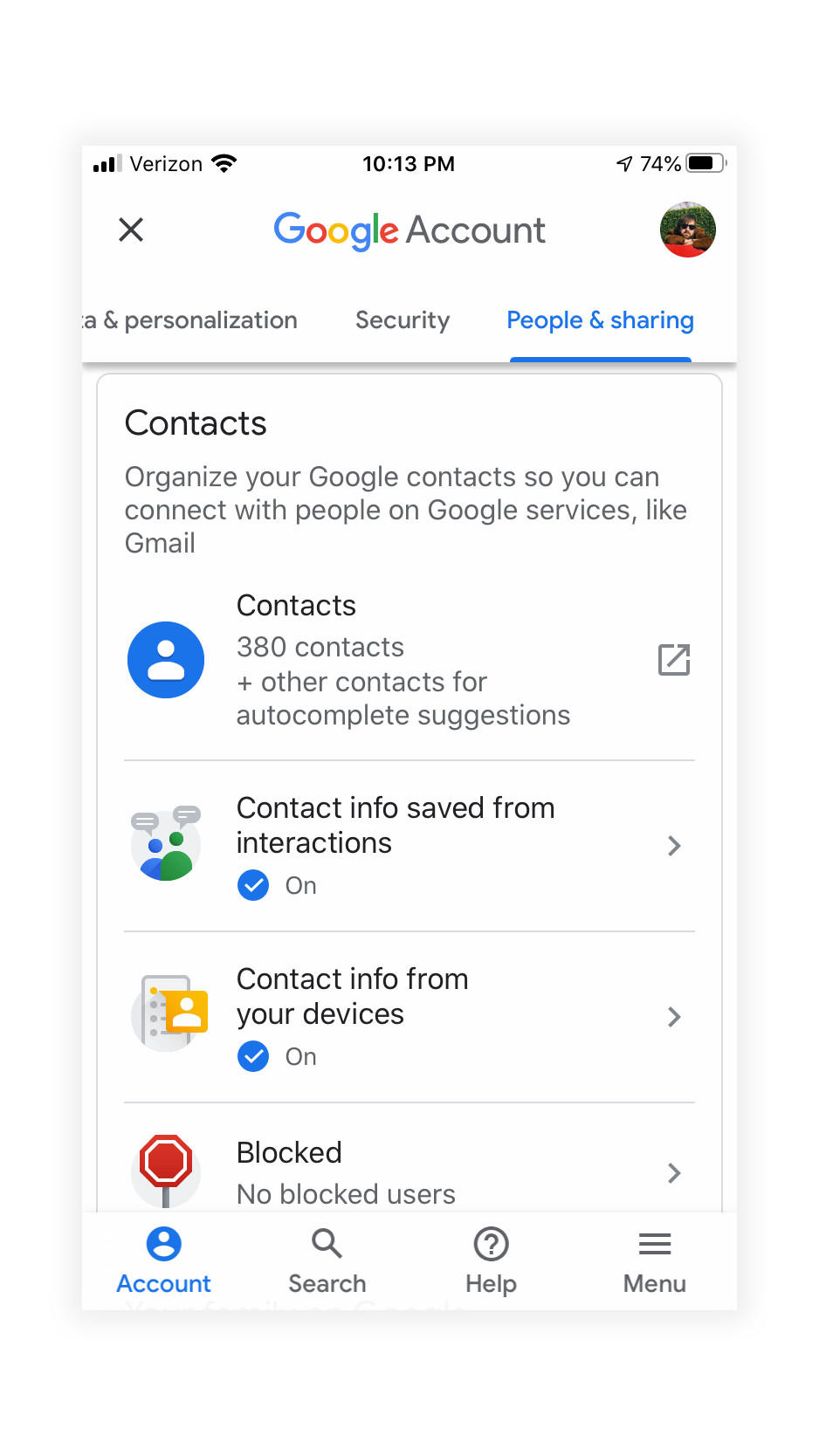The image displays a screenshot from a phone, specifically showing the Google account settings of the user. At the top of the screen, the time is 10:13 PM, and the phone's battery is at 74%. To the right, there is a profile picture of the account owner, who is wearing sunglasses and a brown shirt. The highlighted tab is "People and sharing," indicating the current screen.

The main content of the screen pertains to Google contacts management. It includes a prompt encouraging the user to organize their contacts to facilitate interactions on Google services like Gmail. The user has 380 contacts, along with additional contacts used for autocomplete suggestions. The settings indicate that contact information saved from interactions and devices is turned on. Moreover, there are no blocked users listed.

At the bottom of the screen, several icons are visible, representing different sections, including Account, Search, Help, and Menu. At the top, besides "People and sharing," partial terms for other sections are visible: to the left is "Security," and further to the left, a section partially cut off reads, "...and personalization."